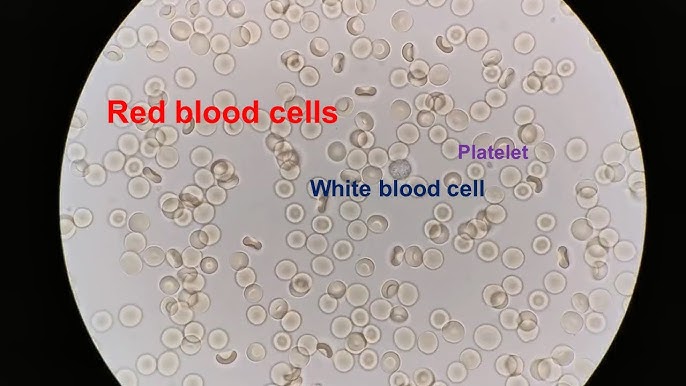This is a detailed illustration resembling a microscope view of blood cells. The central beige area, set against a black background, showcases red blood cells, white blood cells, and platelets. The cells are depicted in varying degrees of clustering, with some flat, some curled, and others spaced out. Red blood cells are highlighted with red text in the top right, while white blood cells appear in blue text in the center, and platelets are denoted in purple text above. The image attempts to mimic the appearance of these components under microscopic examination, with the cells in shades of white and gray within a grayish-blue solution. The illustration is framed in a circular view, reinforcing the perspective of looking through a microscope, though it's ambiguous whether the image is a true photograph or artist's rendition.